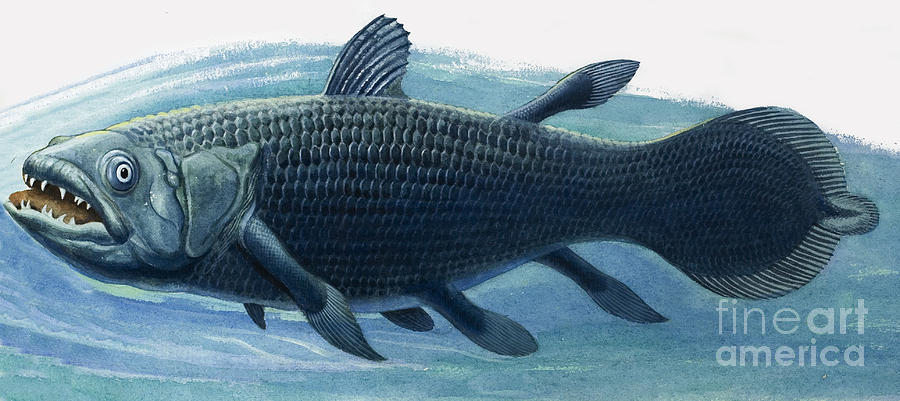This image depicts a surreal, dark grayish-blue fish with an array of ominously sharp white teeth set against a background of swirling blue hues and a stark white upper section. The fish exhibits a variety of vibrant scales and features seven distinct fins along its body, including a unique tail that has an additional circular protrusion. It has a somewhat crazed expression with eyes positioned on either side of its head, and a faded, oven-orange tongue peeking out from its partially open mouth. Though it resembles a catfish or bass, it notably lacks typical catfish whiskers. This unsettling fish artwork is crafted by Fine Art America and immerses the viewer in an eerie underwater scene.